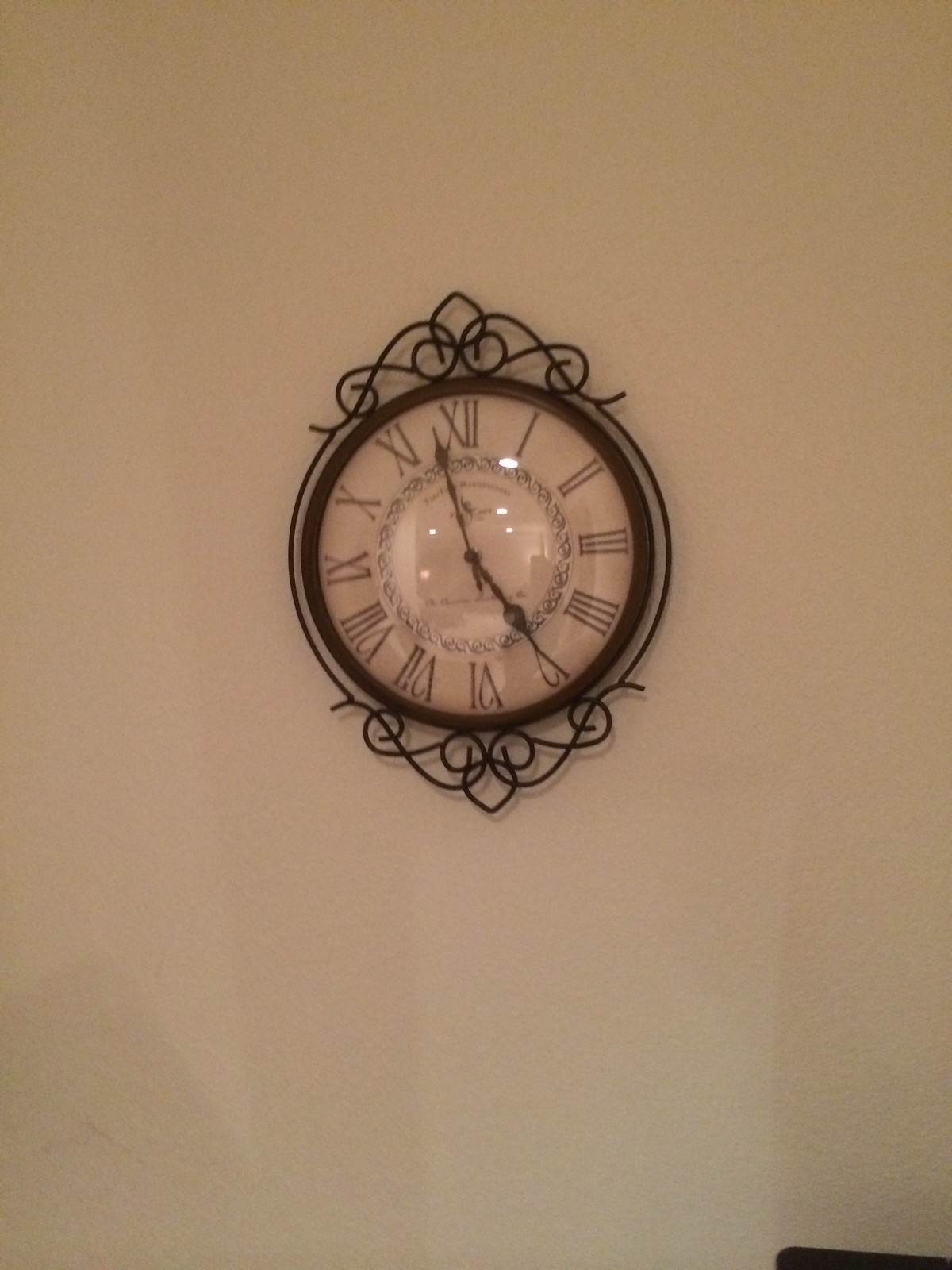A classic, ornate wall clock is prominently displayed against a subtle beige wall, potentially white, enhancing the elegant ambiance of the room. The clock features elegant black numerals and hands, accentuated by a sophisticated black outer frame. Decorative curls embellish the frame, adding a touch of intricate elegance to the piece. The clock's face is a pristine white, creating a striking contrast with the black elements, making it a focal point on the wall. There are no other texts or elements in the photo, emphasizing the clock as a refined centerpiece, likely situated in a cozy and inviting living room or main living space.